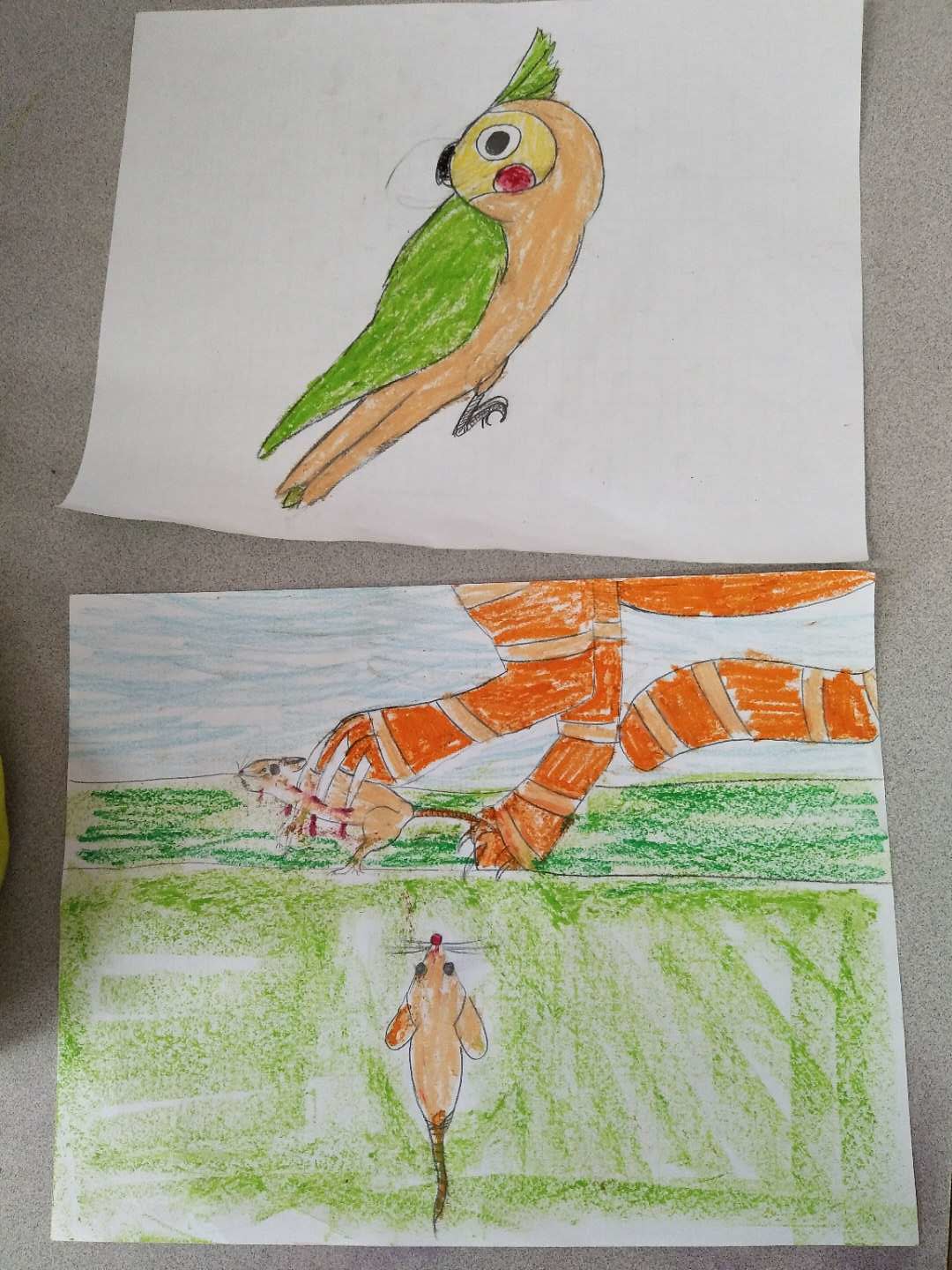This color photograph captures two crayon drawings placed one above the other on a standard grey, speckled plastic-finished tabletop. Both drawings are on standard 8.5" x 11" white paper and appear to be created by children.

The top drawing features a profile view of a small parrot with a distinctively whimsical appearance. This green parrot, with a yellow face and chest, looks backwards over its right shoulder with its head turned. Big, cartoony eyes, marked by round white circles with black pupils and rosy red cheeks, give it an expressive look. Adorning its head are small green feathers, and it has a short black beak. Its black feet are curled up as if perched, although it appears to be floating on the paper.

The bottom drawing depicts a dramatic scene on a largely green crayon-colored field. An orange cat, represented solely by its sharp-clawed front paws and a striped tail extending from the right side of the drawing, is shown gripping a brown mouse, puncturing its body with visible claws. Blood is depicted where the claws enter the mouse's body. Below, a second brown mouse is seen in a top-down view, seemingly witnessing the scene. The use of green crayon dominates the background, dividing into darker and lighter shades, perhaps depicting variations in the grass or ground.

The two drawings, both unsigned, evoke a sense of innocent creativity intertwined with vivid storytelling.